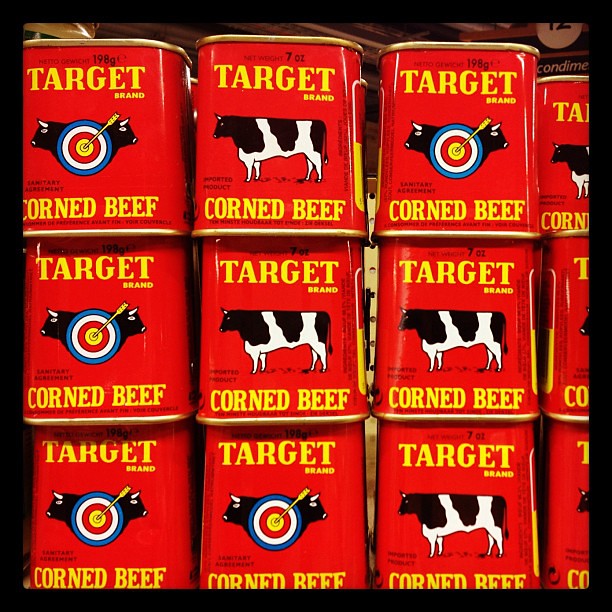This color photograph, likely taken in a Target grocery store in North America, showcases towering stacks of brightly colored, square tins of Target brand Corned Beef that almost completely dominate the image. The tins are predominantly red and feature bold, yellow writing that reads "Target Brand" and "Corned Beef." There are two distinct designs on the tins: one displays a side profile illustration of a black and white cow, while the other features a bullseye target with concentric rings in yellow, red, white, and blue. Two cow heads peek from behind the target, with an arrow piercing the bullseye and pointing diagonally upwards. In the background, glimpses of other products, including a package in dark and light brown, hint at the broader store setting. This scene is punctuated by the repetitiveness of the corned beef tins, underscoring the store's branding and product display strategy.